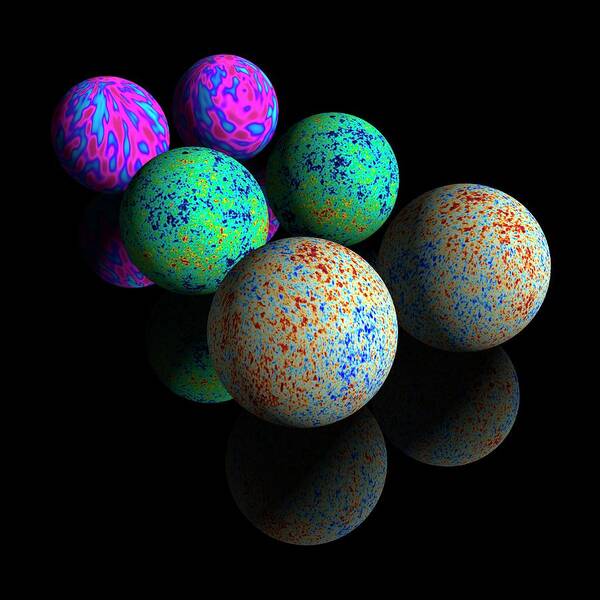This image is a detailed digital depiction of six brightly colored spheres set against a completely black background. Arranged in three rows, the spheres in the back row are predominantly fuchsia with blue streaks and patches, featuring a vibrant heat map-like pattern. Directly in front of these, the middle row contains two slightly larger spheres primarily in lime green with some blue splotches, hinting at a map-like appearance with scattered spots of black, yellow, and red. Lastly, the front row showcases the largest spheres in whitish tones but heavily adorned with mingled brown, orange, beige, red, and blue dots and swirls. The lighting and shading techniques give the spheres a 3D appearance. Reflections of these colorful spheres can be seen on the shiny black surface they rest upon, creating a visually striking contrast. The overall scene evokes the look of artistic, modern jawbreakers set in a meticulously reflective space.